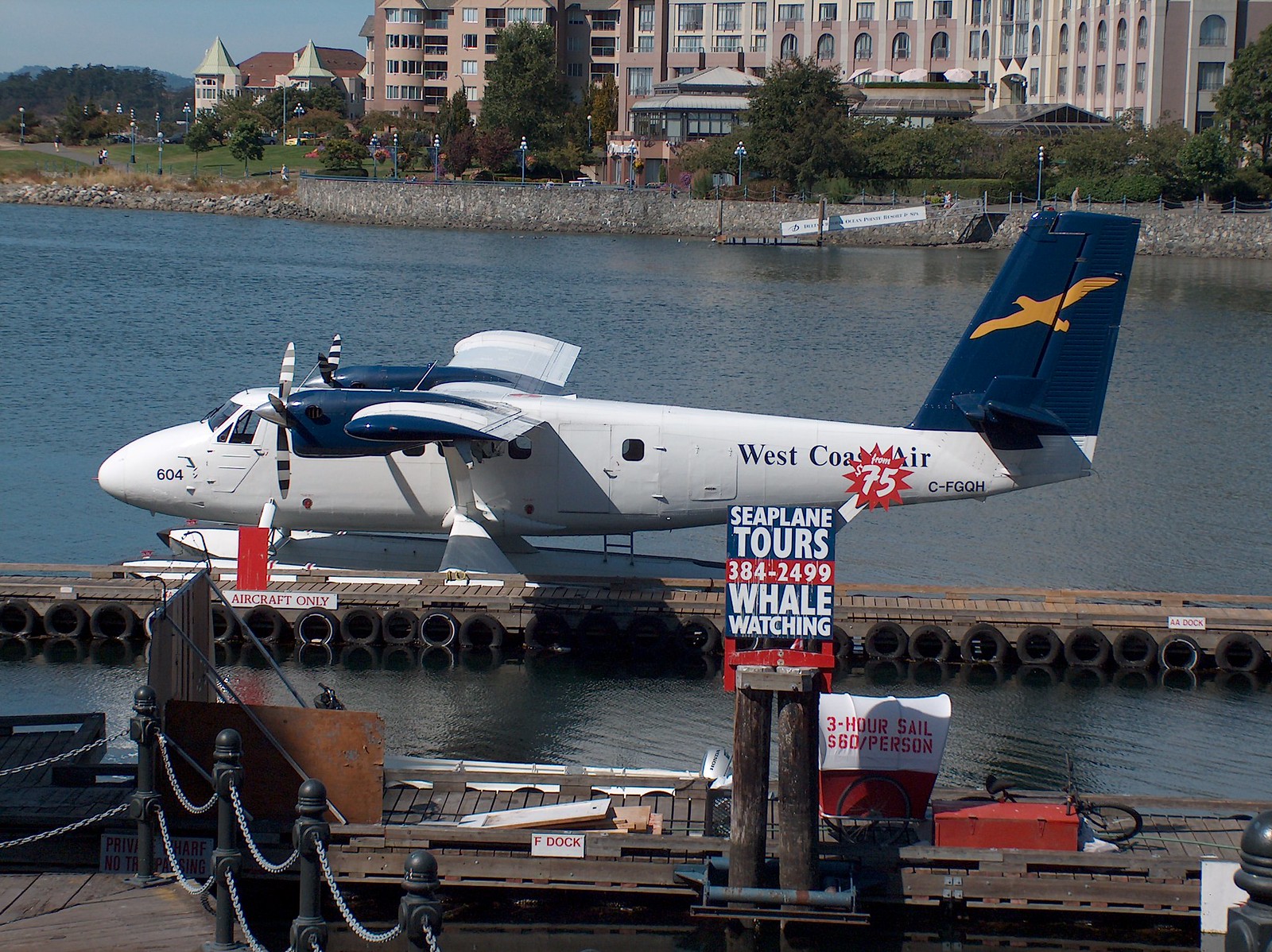The image showcases a bustling seaplane dock with multiple wooden piers extending into a vast body of water. At the forefront, a small seaplane, identified as a West Coast Airplane, is moored. This primarily white aircraft features a distinctive blue fin with a yellow X, black and white striped propellers, and the registration code C-FGO or QH, along with the number 604 on its nose. The plane is equipped with boat-like pontoons, indicating its ability to land on water.

Prominently displayed is a sign advertising "Seaplane Tours," including whale watching tours, with a price of $60 per person for a three-hour trip. The dock it is parked next to is brown and wooden, adorned with black tires along its edge for padding. There is a vibrant mix of signage around, including one in red and white displaying the contact number 384-2499, and another designating it as F-Dock in red letters on a white background.

In the background across the water lies a resort complex, featuring buildings in gray, white, tan, and pink hues, with varied roof colors including brown and light green. The resort area is surrounded by well-maintained green grass, trees, and a pathway populated with strolling visitors. The shoreline near the dock has patches of overgrown yellow grass interspersed with rocks. The clear blue sky stretches above, completing the serene and picturesque scene.